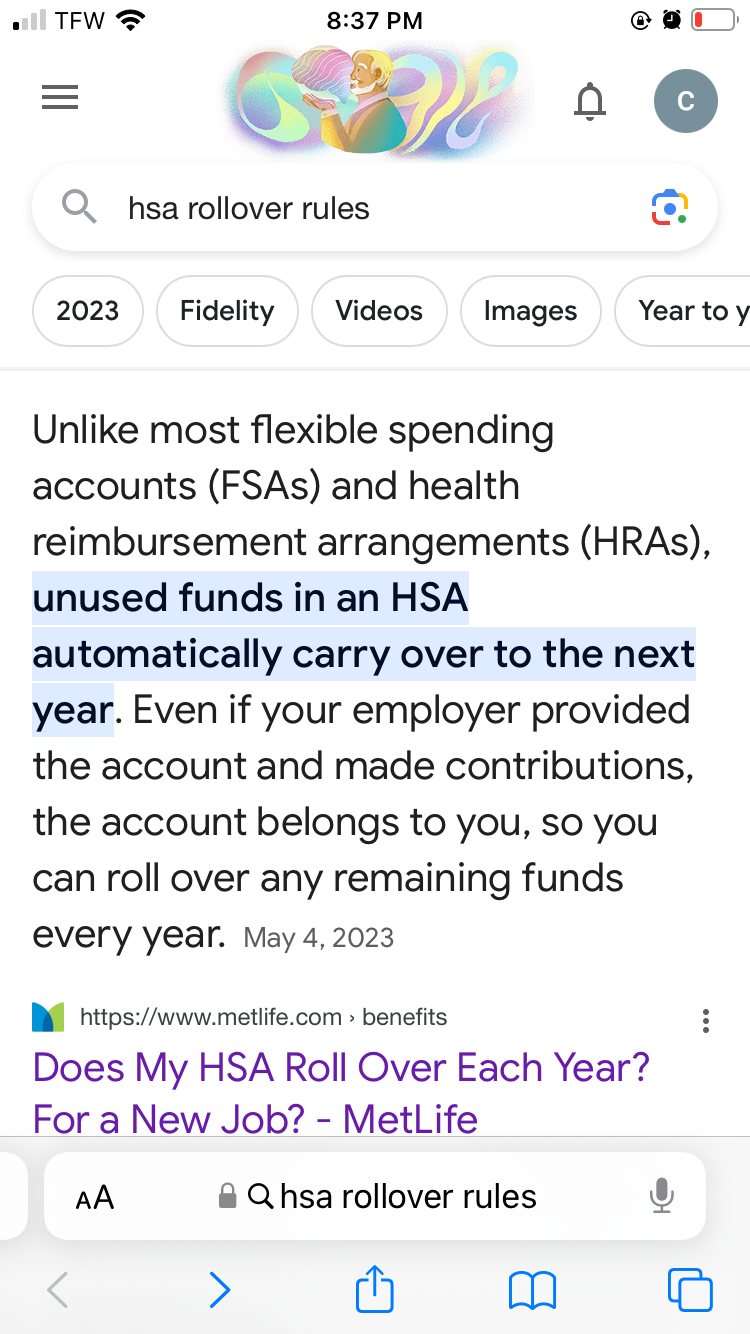The displayed image is a screenshot from a smartphone, framed in a tall, narrow rectangle and featuring a predominantly white background. 

At the top of the screen, various status icons are visible. On the left, there are four bars representing the cell signal strength, with only the first bar being bold. Next to it, the text "TFW" is displayed. In the center, the current time is shown as 8:37 PM. To the right, there are icons for a clock and a lock, followed by a battery icon on the far right, which features a red bar on the left side indicating a low battery level.

Beneath the status bar, there is an image with a swirly, abstract background. In this image, a bearded man is seen in profile with his hand extended outwards. Directly below this image lies a search bar containing the query "HSA rollover rules."

Under the search bar, five response categories are displayed as selectable ovals: 2023, Fidelity, Videos, Images, and Y2Y.

Further down, below the category options, the screen shows search results. The text of the search results is black on a white background, stating:

"Unlike most flexible spending accounts (FSAs) and health reimbursement arrangements (HRAs), unused funds in an HSA automatically carry over to the next year. Even if your employer provided the account and made contributions, the account belongs to you. So you can roll over any remaining funds every year. March 4, 2023."

Certain text in the middle is highlighted with a blue background for emphasis.

Following the informative excerpt, there is a small blue and green icon accompanied by the text:

"https://www.metlife.com care and benefits"

In purple text below, it reads: 

"Does my HSA roll over every year for a new job? MetLife."

Directly underneath, a secondary search bar reiterates the query "HSA rollover rules," this time featuring a microphone icon on the right. The standard smartphone navigation symbols are visible at the bottom of the screen, including left and right carets.